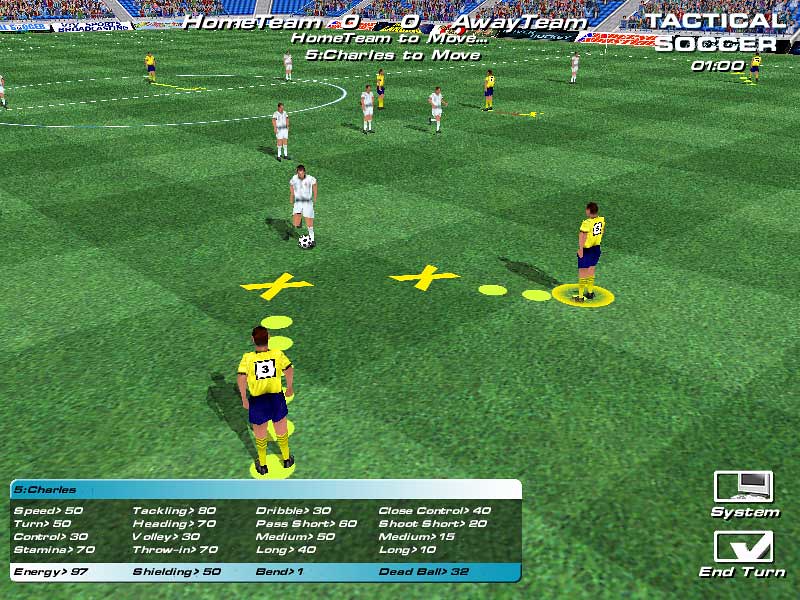This image appears to be a screenshot from a video game titled "Tactical Soccer," which likely dates back to the early to mid-2000s. The image quality is relatively low-resolution, characteristic of that era. The gameplay screen showcases a green field with several players, including two prominently positioned athletes donned in yellow and blue uniforms. The image captures a moment where players are interacting with the ball, illustrating dynamic in-game football action.

Across the top of the screen, the scoreboard displays the current scores for both the home and away teams, with both teams tied at zero. Additionally, there's a timer indicating either one minute or one hour remaining in the game. In the bottom left corner, the interface provides detailed statistics for a player named Charles, including metrics such as speed, control, and turning ability. Finally, the bottom right corner features two buttons labeled "System" and "End Turn," suggesting elements of strategic gameplay where players may need to manage game settings or conclude their turn.